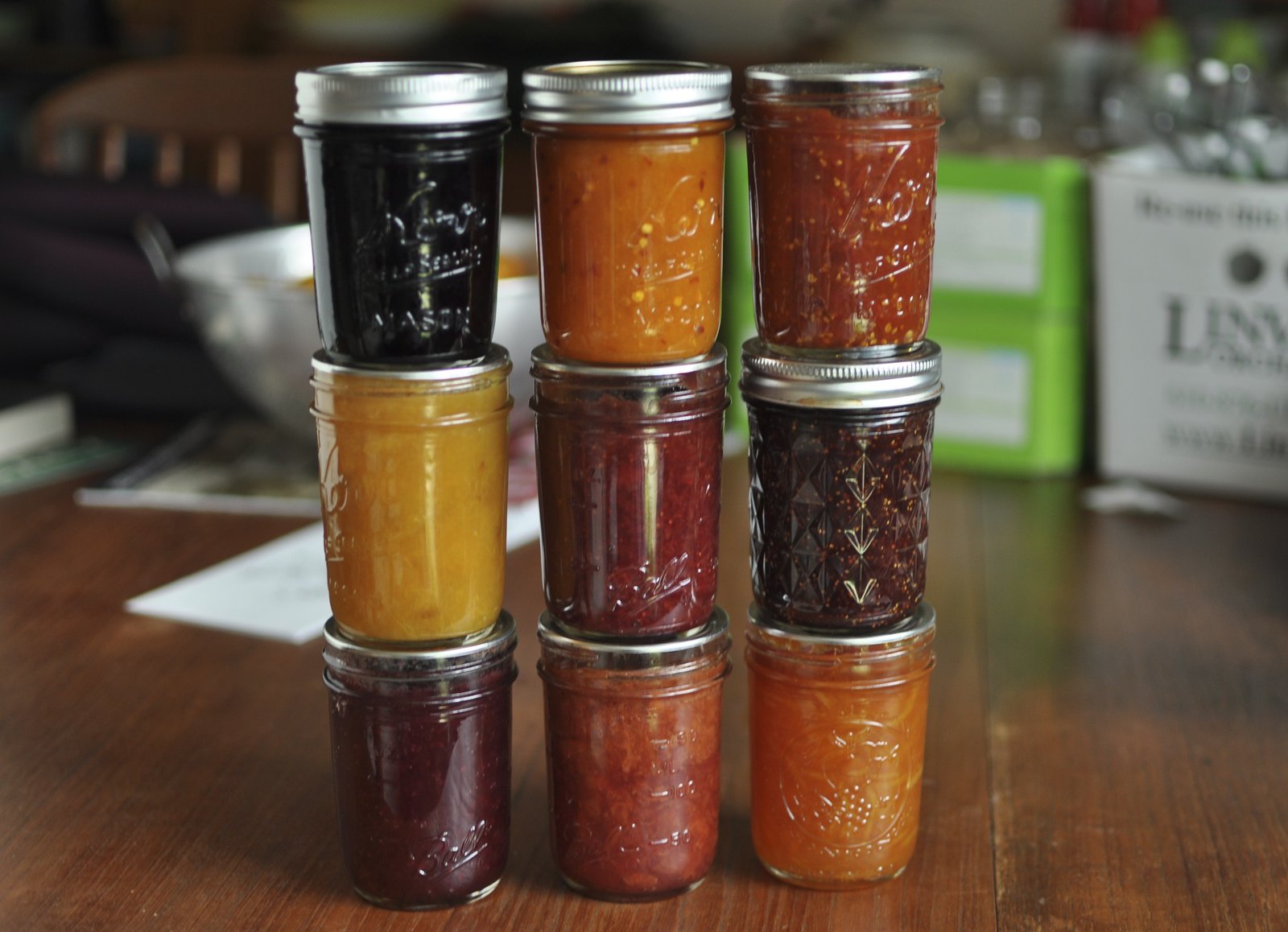The indoor photograph showcases a neatly organized collection of nine small glass mason jars, each with a silver lid, stacked in three rows of three on a wooden kitchen table. These jars, filled with an assortment of colorful jellies and jams, include hues ranging from dark purple, red, light tan, and orange. The jars are intricately detailed, featuring raised lettering on the glass, though it is not legible. In the background, slightly out of focus, there is a large silver mixing bowl to the left and boxes of additional mason jars to the right, adding a sense of depth and context to the jam-making setting.